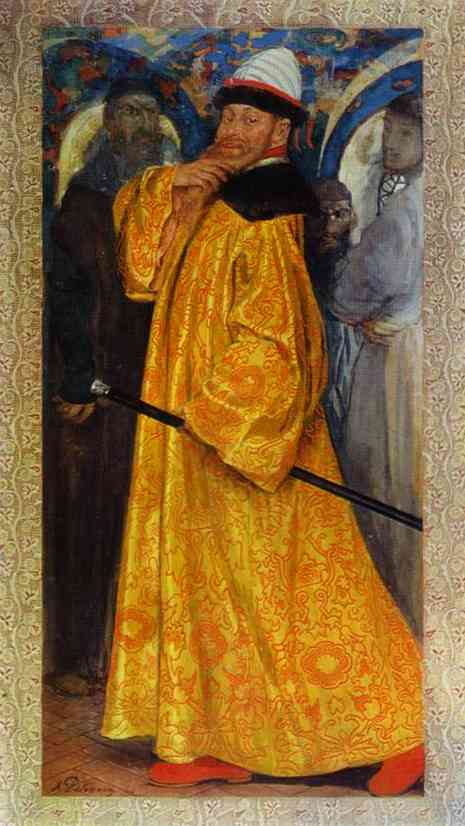This is a detailed, colorful painting titled "The Tsar's Own Fur Line Robe" by Andrei Ryabushkin, created in 1902. The artwork, in portrait orientation, features a man believed to be an Asian emperor or tsar standing in a three-quarter turn towards the viewer. He is dressed in an exquisite, long, flowing gold robe adorned with intricate orange scroll designs, made to look like silk, and a wide black fur collar. The robe extends down to cover his orange shoes. The man sports a slight grin and is touching his red beard with his right hand, giving the impression that he is pondering something. On his head is a distinctive white hat with a blue stripe and a red and black fur brim. In his left hand, held parallel to the ground, he carries a black cane with a silver handle.

The background features intricate details, suggesting an elaborate setting with arched walls adorned in blue, orange, yellow, and gold etchings, possibly reminiscent of a basilica. Two additional figures are present behind the central figure: a man on the left in a long black robe and a tall hat, who has a scowl on his face and is looking straight at the main subject, and a woman on the right in a blue dress, who seems smitten and smiles slightly at him. The floor beneath them is made of red brick tiles. The painting embodies the rich and ornate style of Romanticism.